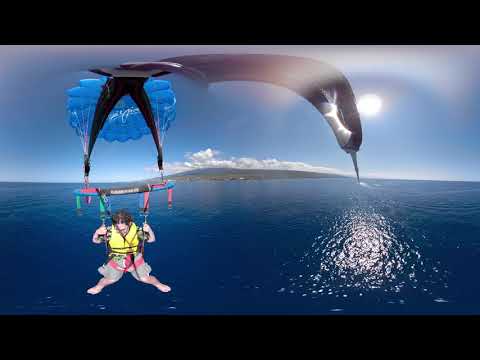The image depicts a striking scene of someone paragliding over a vast, dark blue ocean. The paraglider, dressed in pink trunks and a yellow life vest, hangs beneath a blue parachute accented with green and black, positioned in the bottom left corner of the image. The sea dominates the bottom half of the picture, stretching out to meet a distant island that's centered in the background, crowned with a few white clouds. Above the island, the sky transitions to a lighter blue, with the sun glowing brightly to the right. An intriguing, black object, resembling an ambiguous shape that could be an animal or perhaps a distant diver's legs, is faintly visible near the top of the image, adding an element of mystery. Overall, the scene, with its vibrant colors and surreal elements, evokes a photoshopped aesthetic, blending natural beauty and dreamlike elements seamlessly.